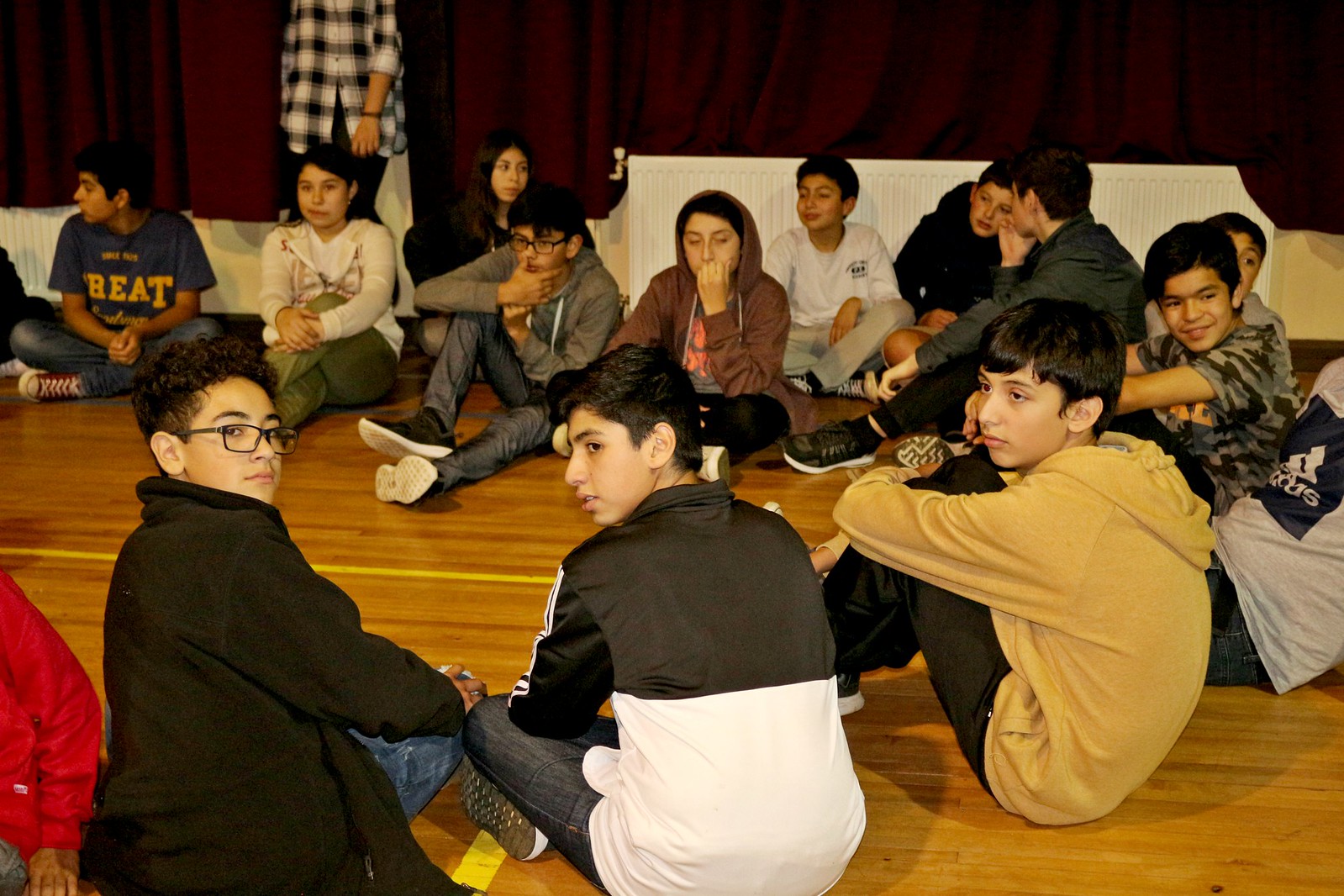In this vibrant color photograph, a group of approximately 12 young middle school kids, around the ages of 13-14, are seated in a circle on a wooden gymnasium floor. Their attire is typical of schoolchildren, featuring various styles such as jeans, sneakers, t-shirts, and long-sleeved sweatshirts. Notably, one boy in glasses is looking back at the camera, sitting next to another boy in a distinctive half-black, half-white shirt. Beside them, another boy donning a camel-colored hoodie gazes off into the distance. The children seem somewhat unimpressed and bored, yet their nice haircuts and smiles suggest they take pride in their appearance. In the background, a woman in a plaid shirt can be seen standing, though her face is obscured. The setting also includes notable features like brown curtains and what appears to be a white furnace, adding context to the roomy gymnasium environment, complete with stage and yellow tape lines on the wooden floor.